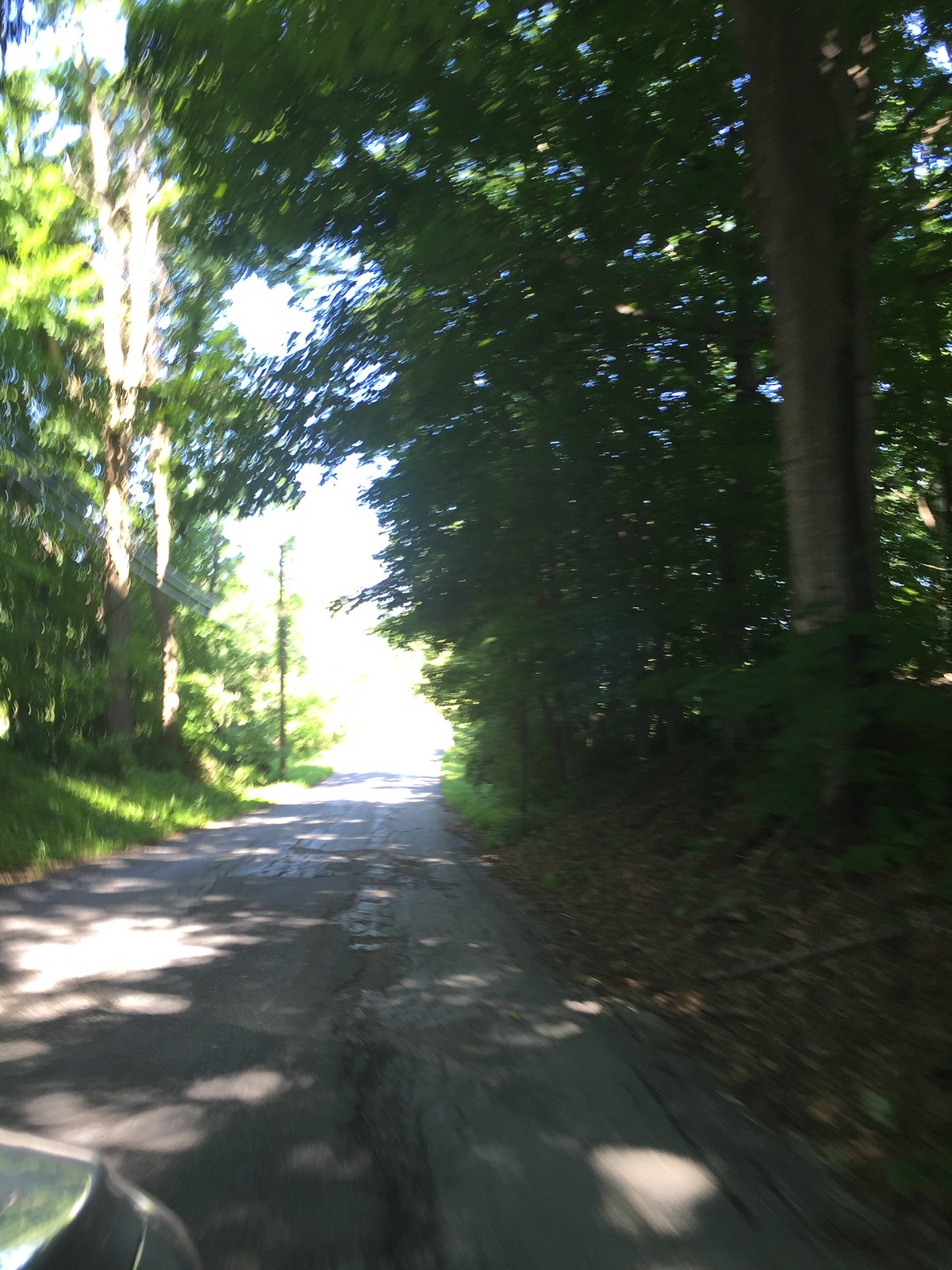A blurred photograph captures the serene essence of a country road, seemingly taken from a moving vehicle, potentially a motorcycle or a car. The road stretches straight into the background, enveloped by a dense, wooded area with towering trees. The tree branches form a natural archway over the pathway, creating a canopy that casts extensive shadows interspersed with bright sunspots where sunlight pierces through the foliage. On the left, additional tall trees are visible, alongside utility poles with telephone wires running parallel to the road. Toward the horizon, the road is brightly illuminated by the setting or rising sun, with patches of clear sky visible through the trees. The ground near the lower right edge of the photograph is scattered with fallen leaves, adding an autumnal touch to the tranquil scene.